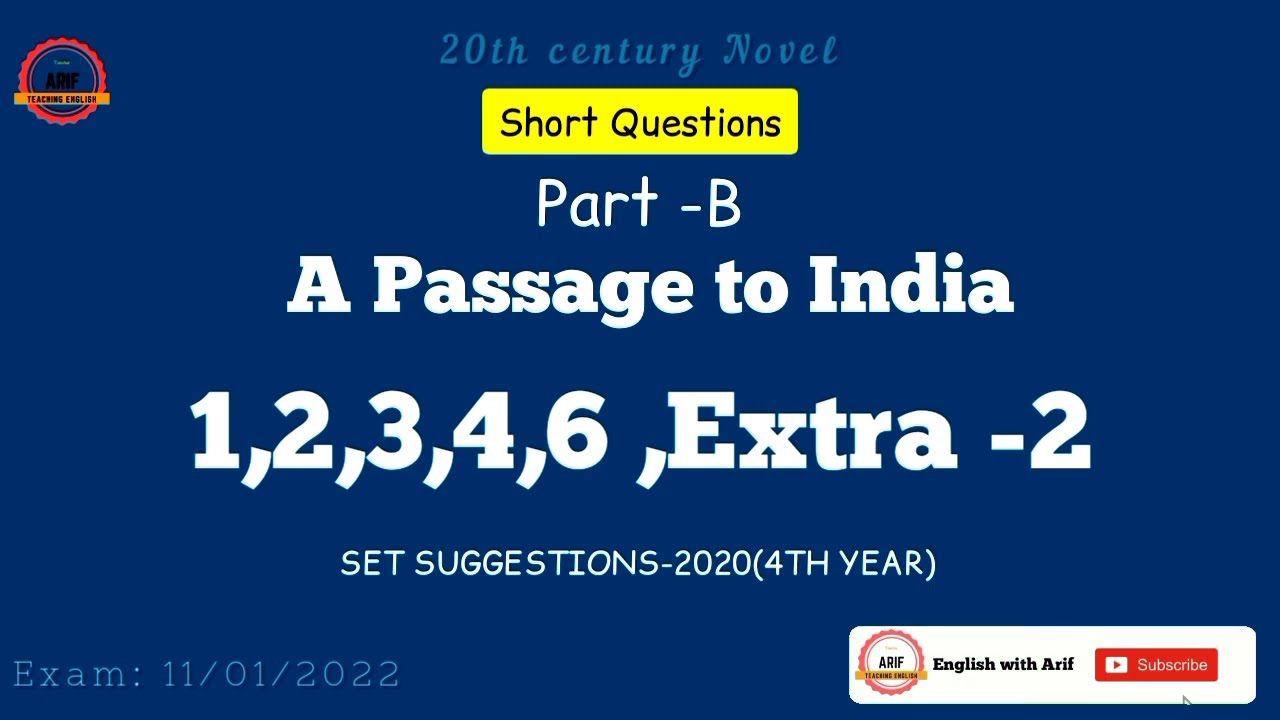The image features a graphic with a medium to dark blue background. At the top, "20th Century Novel" is written in light blue text. Below that, in a yellow rounded rectangle with black text, it says "Short Questions". Further down, in white text, it states "Part-B". Below this, in bolded letters, is the title "A Passage to India". Next, in slightly larger letters, the numbers "1, 2, 3, 4, 6, Extra-2" are listed. Underneath, it says "Set Suggestions-2020 (Fourth Year)". In the lower left corner, the text reads "Exam: 11.01.2022", indicating the exam date. On the upper left, there's an orange logo resembling a gear with a yellow banner that says "Teachers [something]" (the exact words aren't clear). In the lower right corner, against a white background, it says "English with Arif" and includes a subscribe button. This slide appears to be part of a YouTube channel, likely an educational resource for studying English literature, specifically focused on 20th-century novels.